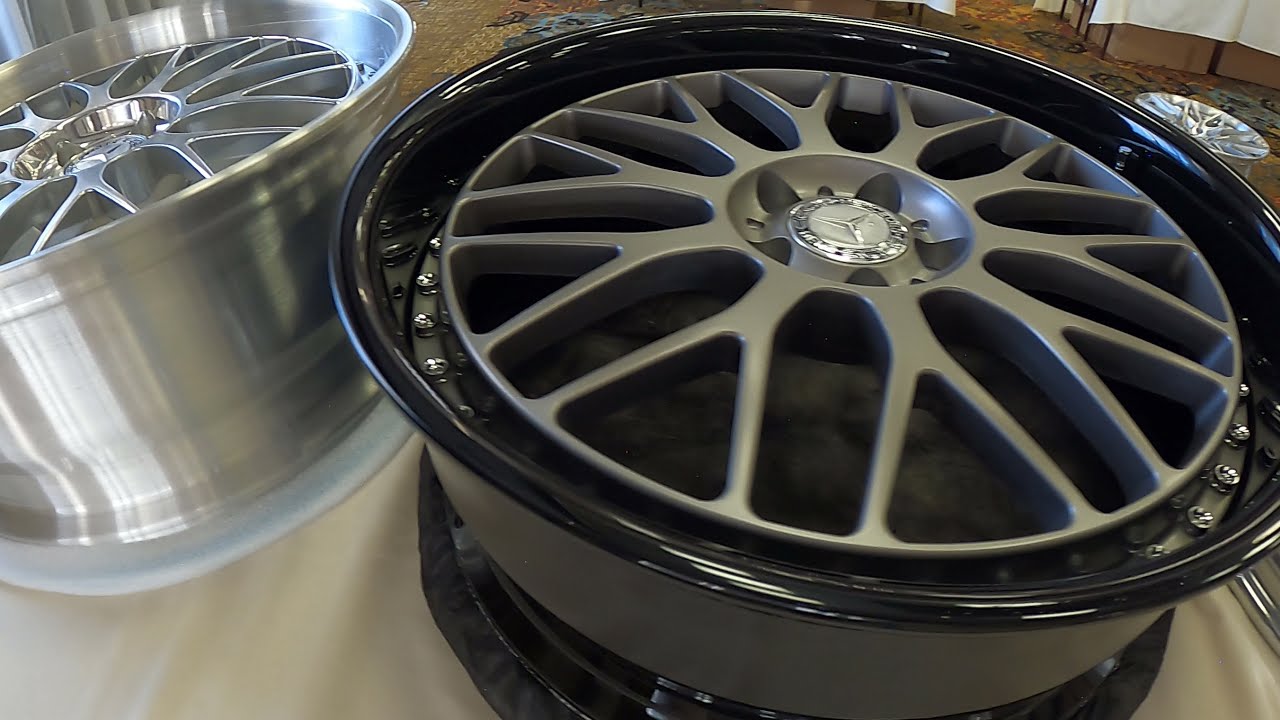The image prominently features two automobile rims displayed on a tabletop covered with a white tablecloth that is just visible beneath them. The central focus is a black Mercedes-Benz rim positioned slightly to the right of center. This rim has a gray center with silver spokes radiating from it, showcasing the Mercedes logo at its core. To the left, almost at the top left of the image, is another rim that is entirely silver, sharing a similar spoke design but with no visible logo. In the distant background, towards the top right, there is a faint glimpse of another silver rim. The rims appear elevated, likely placed on a table as part of a display. The backdrop reveals additional tables covered with white tablecloths and hints of boxes underneath, contributing to the setting. The floor features a carpet with patterns of green, red, and yellow, enhancing the room's detailed decor. Nevertheless, the black Mercedes-Benz rim remains the photograph's primary subject, with the silver rim offering a complementary contrast.